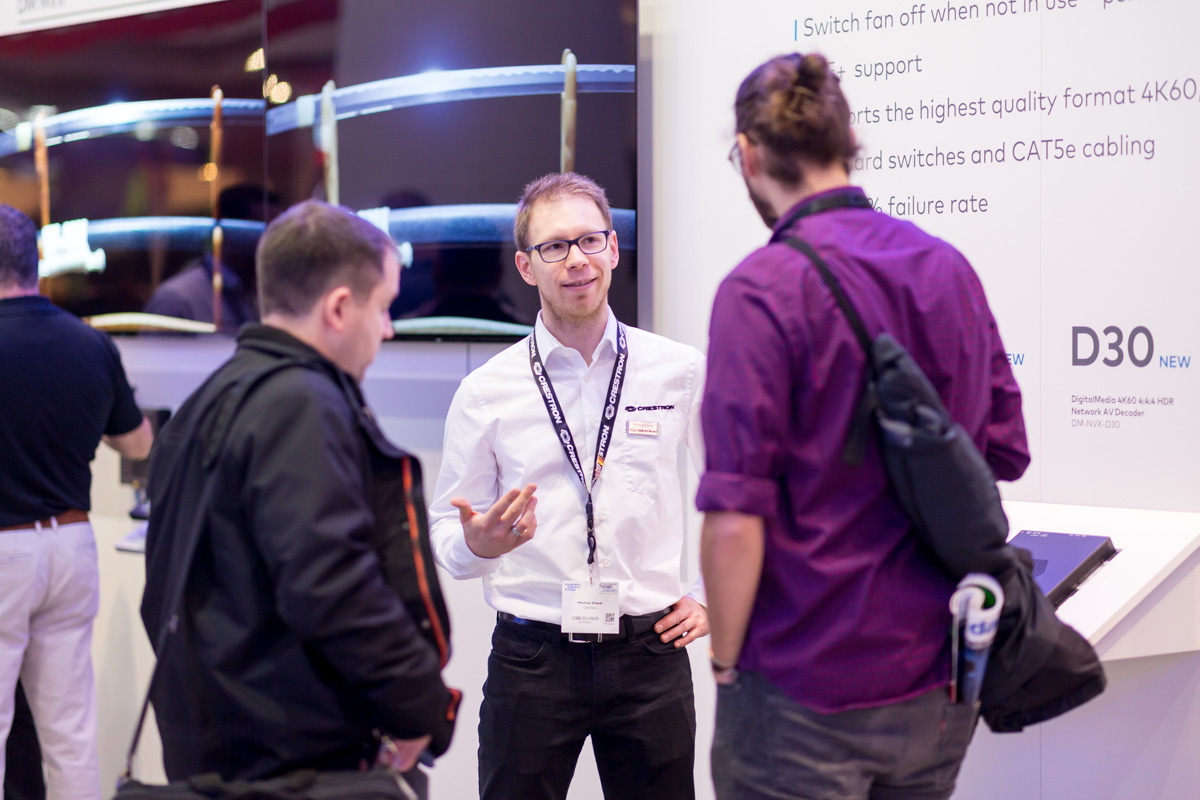The image depicts three young men engaged in conversation in a bustling exhibition hall. Positioned in the center, a man wearing a white shirt, black pants, and a lanyard with an ID is facing the camera. He has short brown hair, dark-rimmed eyeglasses, and is gesturing with his right hand as he speaks. To his left is a man in a black jacket with short brown hair, a shoulder bag, and blue jeans with a magazine rolled up in his right rear pocket. To his right is a man with dark hair pulled back in a bun, wearing a purple shirt with rolled-up sleeves and a black shoulder bag slung over his left shoulder. Behind them, there is a white poster displaying partial text related to technical specifications, including terms like "highest quality format," "four K," and "CAT five E cabling." Additional exhibition attendees and display counters can be seen in the background, contributing to the dynamic atmosphere of the scene.